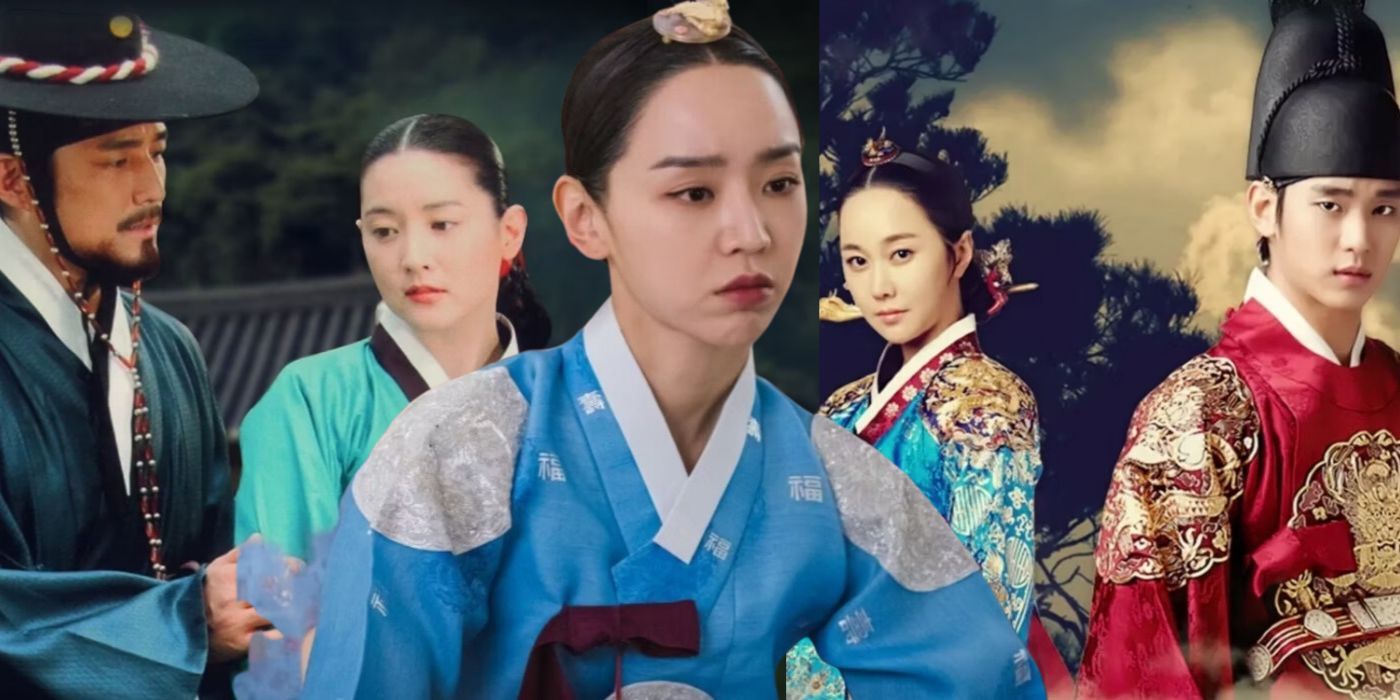This promotional photograph, likely for a traditional Chinese television show or movie, features five characters poised in a serious and thoughtful tableau. At the forefront and center stands a young East Asian woman with a troubled expression, donned in a simple blue kimono adorned with white lettering. Her hair is elegantly pulled back, topped with a decorative flower. Flanking her are two female characters. To her immediate right is a woman in a teal kimono with a blue, white, and gold patterned design, her hair similarly styled with a middle part. To her left is another woman, appearing more subtly adorned, but both maintain the same solemn expression. The two men bookend the group; the man on the far right is striking in an ornate red kimono richly decorated with gold, and he wears a traditional black conical hat. Contrasting him, the man on the far left is dressed in a black robe and a black, wide-brimmed hat reminiscent of Western styles, adorned with a red and white braided cord draped around the brim, and sports a goatee and mustache. Behind this ensemble, the backdrop reveals muted trees and a cloudy sky, adding an atmospheric depth to the evocative scene.